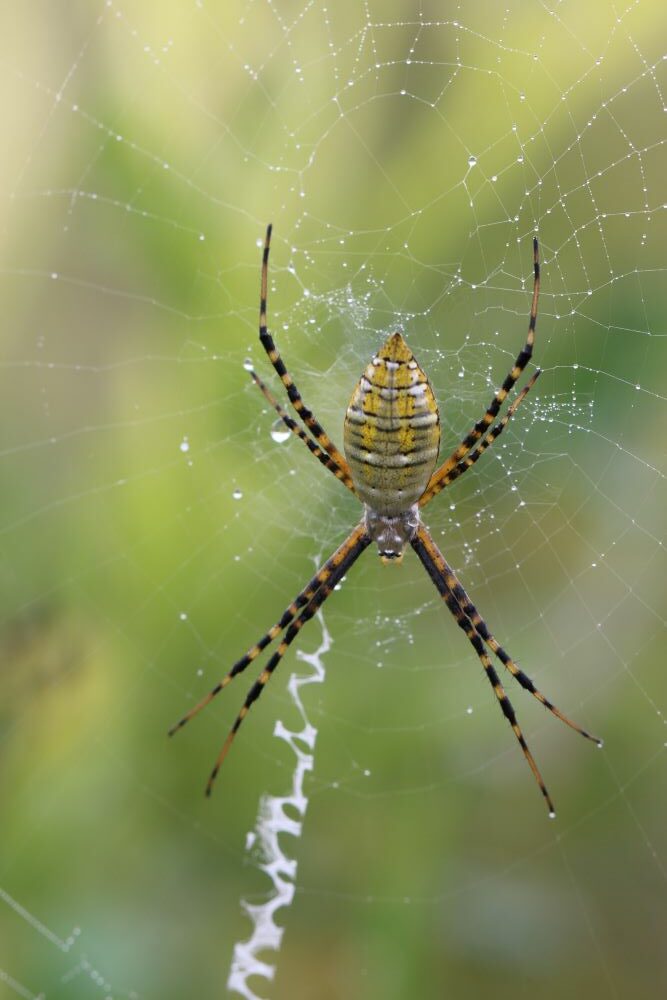This close-up image showcases an intricately woven spiderweb with the background beautifully blurred in shades of green, yellow, brown, and tan. At the center of the web sits a spider, seen from a top-down perspective, displaying its distinct, patterned body and eight legs. The spider's legs are long and thin, adorned with striking black and yellow stripes, and are occasionally grouped together, making them appear fewer in number. Notably, spines line each leg, adding to their detailed appearance.

The spider itself features a body with a gradient of colors starting with a silvery head that transitions into yellow and black toward the pointed end of its abdomen. The pattern resembles horizontal stripes or squares in white, yellow, and outlined black. The spider's large abdomen may suggest it's carrying eggs. Near the spider and extending from the web's center to the lower left, thicker webbing is visible, providing additional texture and complexity to the web.